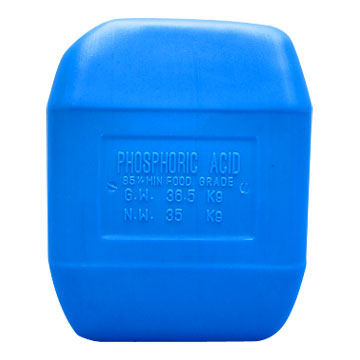The image depicts a small, blue, rectangular plastic container floating against a stark white background, creating the illusion that it is suspended in a white void. The container, which resembles the size and shape of a dental floss container with rounded edges, appears to be a single molded piece of plastic with no discernible top or bottom. It features raised lettering within a recessed rectangle in its center, indicating it is specifically designed to store phosphoric acid. The lettering reads: "Phosphoric Acid, 85% Min Food Grade, GW 36.5 K9, NW 35 K9."